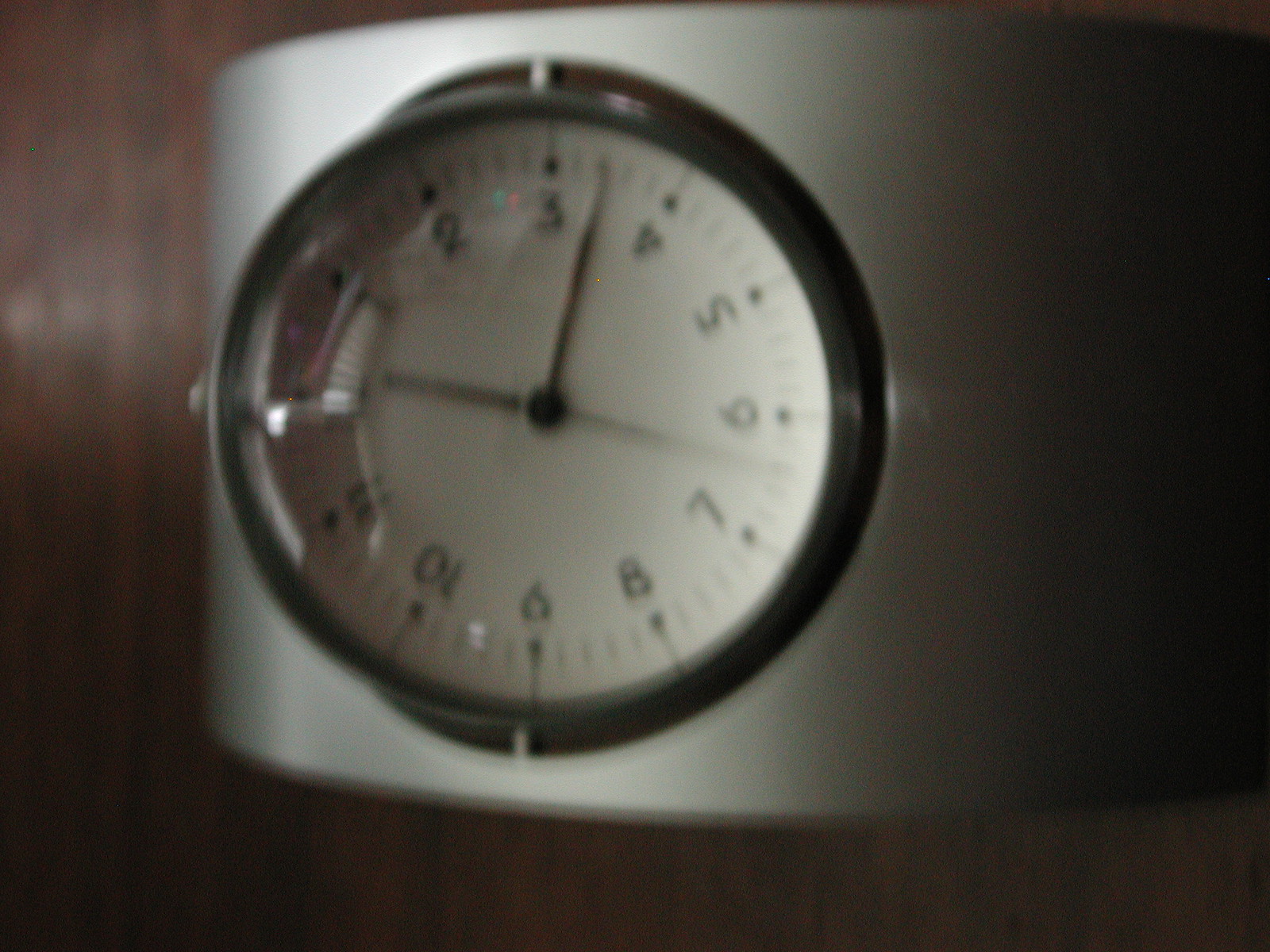This image features a blurry clock that seems to be hanging on a wall or positioned on a tabletop with a brownish backdrop. The clock appears to be rotated 90 degrees to the left, with the "12" positioned where the "9" should be. Encased in a thin black frame, the circular clock has a white face adorned with black Arabic numerals from one through twelve. Each numeral is accompanied by a short line ending in a black circle, and there are rectangular tick marks between the numbers. The hands, including a second hand, are all black. There is a reflection visible on the left side of the clock face, though the source of the reflection is indeterminate. The clock is set in a gray or silver, rounded surface with a hole where the clock face sits. The time displayed is just after 12:17. The clock also seems to have a glass covering over its face.